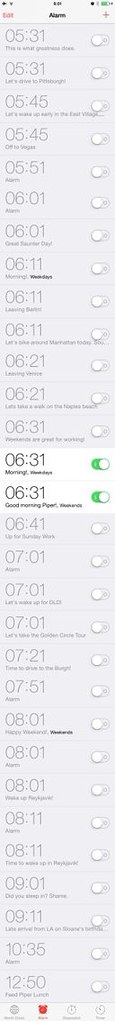The image is a detailed screenshot from a mobile alarm clock app, meticulously stitched together to show a long vertical list of alarm settings spanning from 5:31 AM to 12:50 PM. At the top left, a red "Edit" button is visible, with "Alarm" written in black at the top center, and a red plus sign on the upper right. The status icons like the battery meter and other phone type icons are also visible along the top edge. The list comprises around 30 alarm times, predominantly greyed out indicating they are turned off. However, two alarms set for 6:31 AM stand out with black text on a white background and their sliders toggled to the right, revealing a green indicator showing they are active. These two alarms include labels: one mentions "morning weekdays" and the other "good morning, Piper, weekends", suggesting custom messages for different days. A distinctive red alarm clock icon is situated at the bottom of the list.